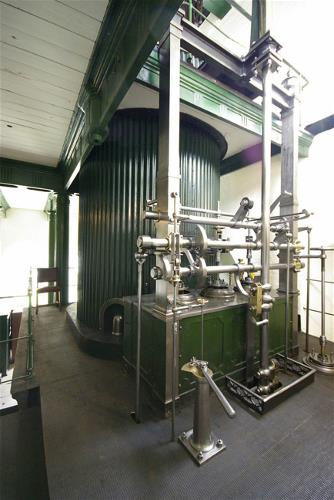The image captures a detailed scene inside a factory, focusing primarily on a large industrial mechanism. We are positioned on an elevated platform enclosed by a railing, with a couple of steps leading down. The platform, possibly made of slate, offers a clear view of the machinery. Centrally located is a massive cylindrical drum, dark gray in color, featuring vertical ridges along its surface.

This sizable drum, which might be used for manufacturing processes such as brewing (though this is uncertain), is surrounded by a network of metal pipes and tubes situated both vertically and horizontally. Directly in front of the drum are several gears and mechanisms, along with a prominent silver handle, which are likely involved in regulating the drum's operation.

The machinery exhibits a blend of gray and green hues, with some green metal paneling visible on different parts. Towards the front of the image, a green box or cabinet with a stainless steel top is noticeable at the bottom, connecting various pipes to the floor. In the background, there’s a second level or ceiling area visible on the upper left side. Additionally, a chair can be seen in the distance on the left-hand side of the platform, contributing to the intricate industrial setting.